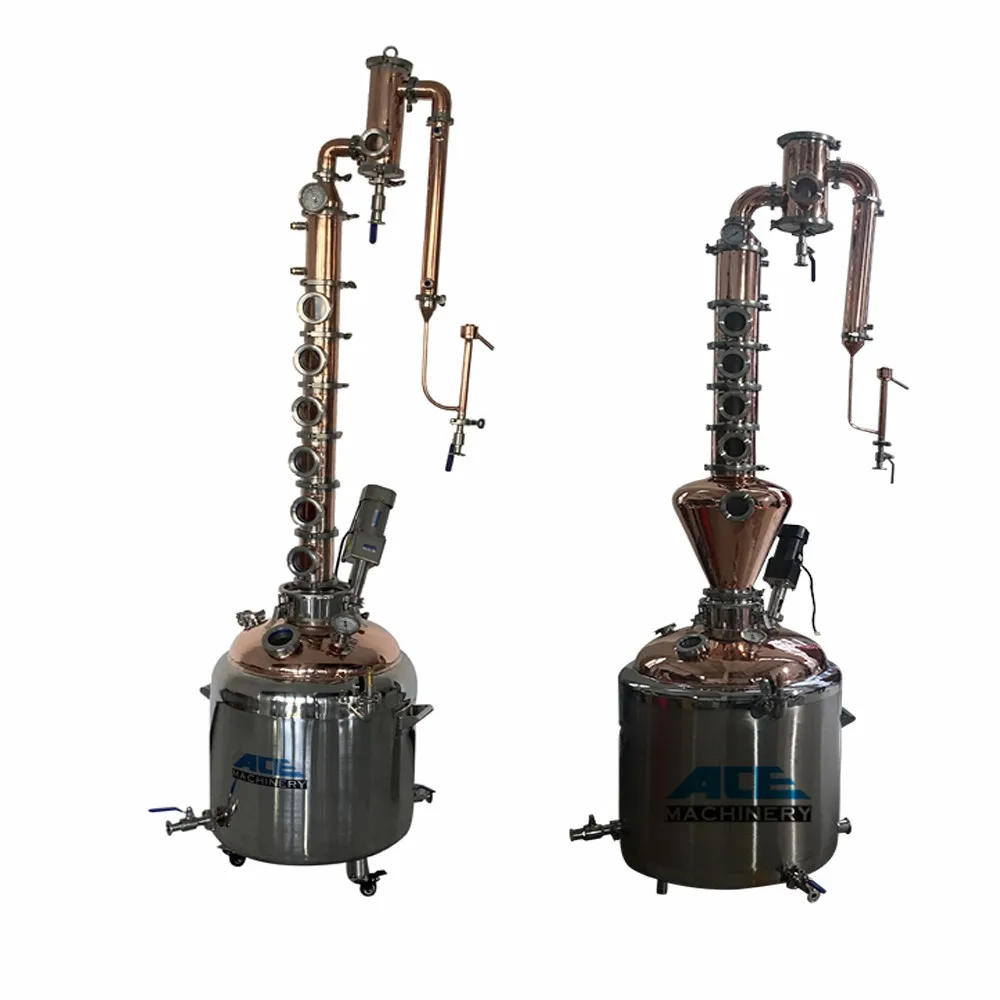The image features two pieces of industrial equipment, prominently labeled "Ace Machinery" with the logo in blue and black lettering. These machines are side by side, and both have a similar design. Each features a round, flat-topped silver tank as its base. From this base, a vertical brass pipe with multiple circular openings runs upward. At the top, the pipes extend horizontally to the right before hooking downward. Both machines are intricate and appear to be entirely made of metal, indicating their likely use in a pressurized system. Valves and additional connected pipes suggest complex functionality, extending likely into other equipment or the wall. The taller machine is situated on the left, with its smaller counterpart on the right.